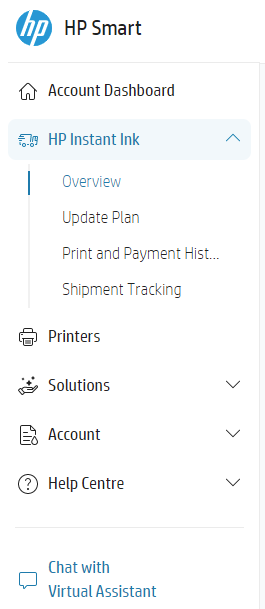Screenshot of the HP Smart Interface:

The screenshot captures the interface of the HP Smart application, showcasing a segment of a page or a window. At the very top, a blue HP icon is prominently displayed next to the text "HP Smart." The background is a clean, white canvas, with all text presented in either black or blue for contrast.

From the top of the interface down, the layout is as follows:
1. **Home Icon**: Accompanied by the label "Account Dashboard."
2. **Truck Icon**: Depicting "HP Instant Link," which is currently blue and highlighted, indicating it's an active selection.
   
   Underneath "HP Instant Link," a submenu is expanded with:
   - "Overview" in blue text.
   - "Updated Plan," "Print and Payment History," and "Shipment Tracking" all in black text.

Returning to the main menu, additional options include:
- **Printers**
- **Solutions**
- **Account Help Center**

Each of these main menu items features a down arrow to their right, signifying expandable sections for more detailed information.

Finally, at the very bottom of the page, there's an option labeled "Chat with a Virtual Assistant" in blue text, paired with a universal instant messaging bubble icon to its left.

Overall, the design is minimalistic and clean, focusing on ease of navigation and readability.